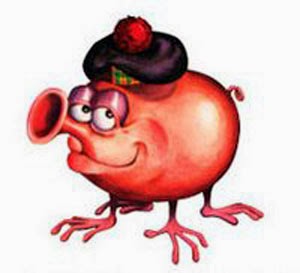The image depicts a peculiar cartoon character with a bulbous, elongated body that resembles a piggy bank but is more red than pink. At the rear, it has a curly tail akin to a pig's, and it stands on four leg-like appendages that resemble frog’s legs, each ending in four toes. The character's head features large, heavy-lidded eyes, giving it a somewhat knowing and smug expression as it gazes upward and slightly to the left. Atop its head is a traditional Scottish hat, characterized by a yellow and green plaid pattern with a red fluffy ball on top, and a black band beneath it. The character’s nose is an unusual feature: it looks like the end of a bugle or a vintage bicycle horn, with a circular opening and a tube extending down to the mouth, which forms a subtle smile. The creature's overall appearance is rounded and glossy, suggesting it might be reflecting light, and it’s set against a stark white background.